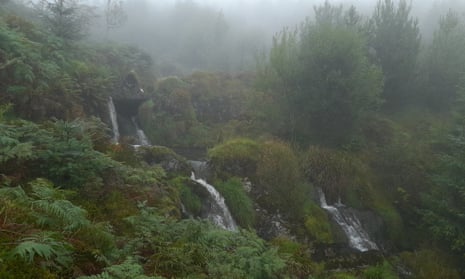The photograph captures a lush, mist-covered landscape featuring multiple waterfalls cascading down a cliffside, part of which is obscured by a dense array of plants, rocks, and green foliage. The scene is characterized by its wild, overgrown appearance, with a variety of shrubs, moss, and algae clinging to the rocks. Majestic, leafy green trees, including some that appear to be evergreens or pine trees, fill the background, adding to the dense, tropical-esque atmosphere. The pervasive mist and fog create a hazy, humid ambiance, rendering the distant trees and other vegetation less distinct. This natural, untamed area, possibly located in regions like Oregon or Washington, exudes a serene, untouched beauty with muted colors that enhance its tranquil, verdant charm. There are no signs of civilization, emphasizing the pristine wilderness of the scene.